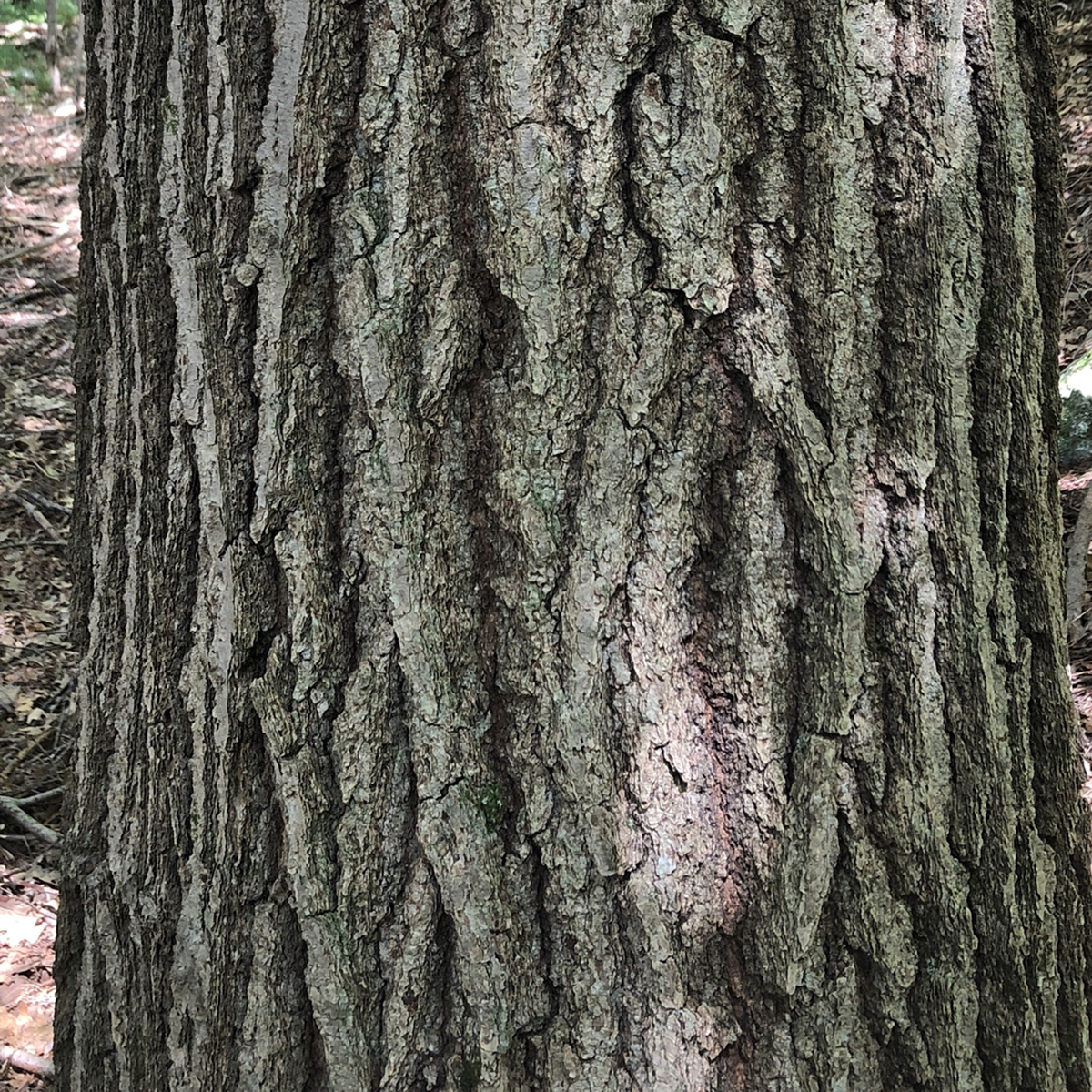This detailed close-up photo captures the thick, deeply grooved trunk of what appears to be an oak tree, primarily at its base. The ground surrounding the tree is strewn with sticks, tree bark, and dirt, with very little greenery visible, suggesting an outdoor setting likely at the base of a hill. The trunk's bark is rich in color and texture, marked by greenish-brown hues and contrasted by patches of thickly covering moss, lending it a varied appearance. Towards the bottom right of the image, a discolored knot hole is visible, featuring a tan left side, green top and right sides, and a brown crease dividing these colors. Notably, there is an unusual pink patch on the trunk that resembles pink powder, possibly indicating a fungal infection or infestation.